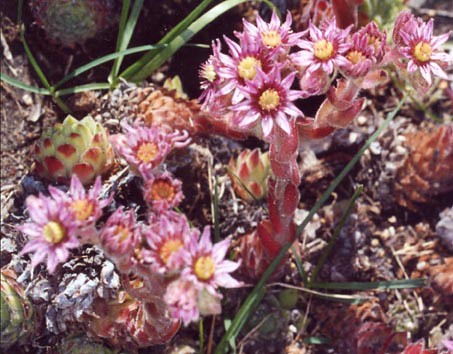The image captures a vibrant outdoor garden scene under sunny skies, featuring a variety of succulent plants and flowers. Central to the composition are clusters of succulents, some of which boast a green base with red-tipped leaves, and others that exhibit a unique pink hue. These pink succulents are adorned with teardrop-shaped petals, encircling yellow centers with a ring of pinky-red. Interspersed among these are grass shoots and a tall, vertically-growing succulent with a red body. Additionally, there are plants with a green artichoke-like appearance, tipped with purple. The soil, visible in the background, is a rich brown, contributing to the earthy palette of the scene. The photo, taken with a slight blur and zoomed in focus, seems to have captured a small, colorful square of a garden, teeming with a diverse array of plant life.